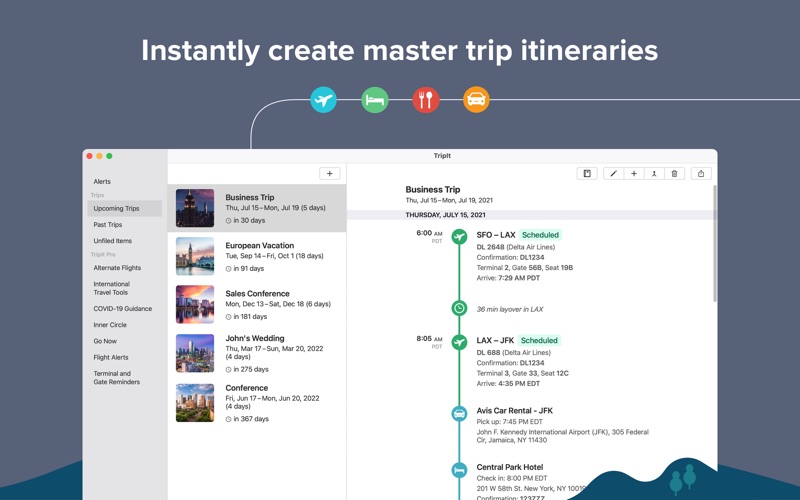**Caption:**
The image is a detailed screenshot of an advertisement for a trip itinerary management company, prominently featuring a minimalistic gray background. Centered at the top, the ad states, "Instantly create master trip itineraries." A line connects a MacBook screen on the left to various icons representing travel components like a car, restaurant, bed, and airplane.

The MacBook screen showcases the Trip It application. The top left corner of the screen includes navigational buttons, and on the left-hand side, multiple alerts and categories are listed, including: upcoming trips, past trips, unfiled items, alternate flights, international travel tools, COVID-19 guidance, Inner Circle, Go Now, flight alerts, and terminal and gate reminders.

The center of the screen displays a list of trips with accompanying pictures: a business trip, a European vacation, a sales conference, John's wedding, and another conference. The highlighted trip, a business trip from Thursday, July 15th to Monday, July 19th, 2021, reveals detailed information on the right.

The business trip details specify:
- **July 15th:**
  - 6:00 AM: Flight from SFO to LAX (Delta), Terminal Arise 729, duration with a 36-minute layover.
  - 8:05 AM: Flight from LAX to JFK (Delta), arriving at 4:35 PM EDT.
  - 7:45 PM: AFIS car rental pickup at JFK.
  - 8:00 PM: Check-in at Central Park Hotel, address provided.

The layout, icons, and comprehensive trip information illustrate the application's capability to organize and streamline travel plans efficiently.